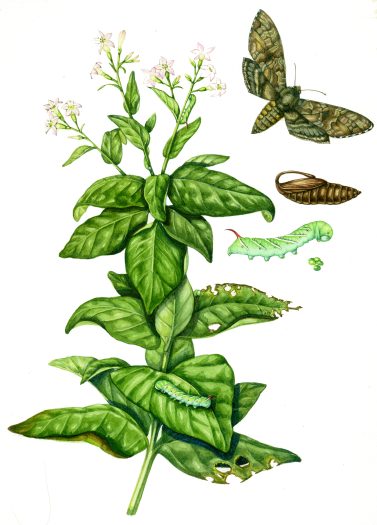This detailed illustration depicts the life cycle of a butterfly, set against the backdrop of a flowering plant that resembles an indoor ivy with its deep green leaves. The scene is rich with botanical detail, capturing the plant's lush, leafy bottom and its delicate pink flowers at the top. Caterpillars are seen munching on the leaves, evident from the holes left behind. To the side, a small green caterpillar is shown in its initial stage, progressing to a much larger, plumper caterpillar further up the plant. Above this, a brown cocoon is depicted, marking the next stage in the transformation. At the topmost point, a butterfly, almost camouflaged against the floral backdrop, emerges from the cocoon, newly transformed and seemingly about to take flight. This comprehensive visual is perfect for educational purposes, such as in biology or science textbooks, catering to a broad audience from elementary to college students.